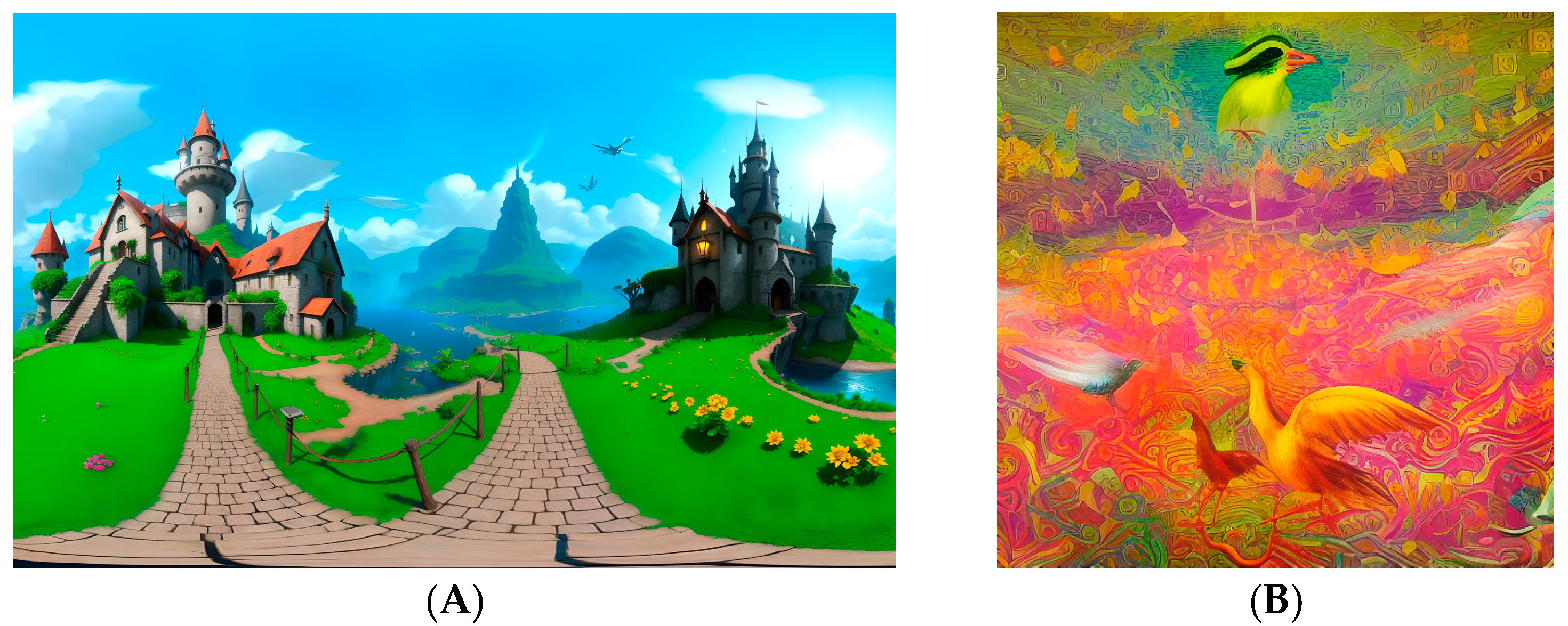This composite image features two distinct scenes, each labeled "A" on the left and "B" on the right. Image A presents a fantasy setting with two different castles. The first castle, positioned on the left, is a grand stone structure with red roofs, featuring several turrets and towers, and set amidst a pleasant landscape. A pathway in the foreground leads towards another path that winds into the distance, eventually reaching blue-tinged mountains in the middle background. Yellow flowers dot the green grass surrounding this castle, and the sky above is a serene light blue with scattered white clouds.

In contrast, Image B on the right offers a surreal, psychedelic vision. This scene depicts another castle, similar in structure but with an ominous atmosphere overshadowed by darkness. The castle is illuminated only by a solitary torch at its entrance, casting long shadows. The entire composition is awash with vibrant, contrasting colors—bright pinks, oranges, greens, and yellows creating a dreamlike setting. Birds, prominent in their colorful display, are scattered throughout, with one bird centrally positioned at the top, looking to the right. The image is dominated by swirling patterns and vivid color schemes, lending it an ethereal quality.